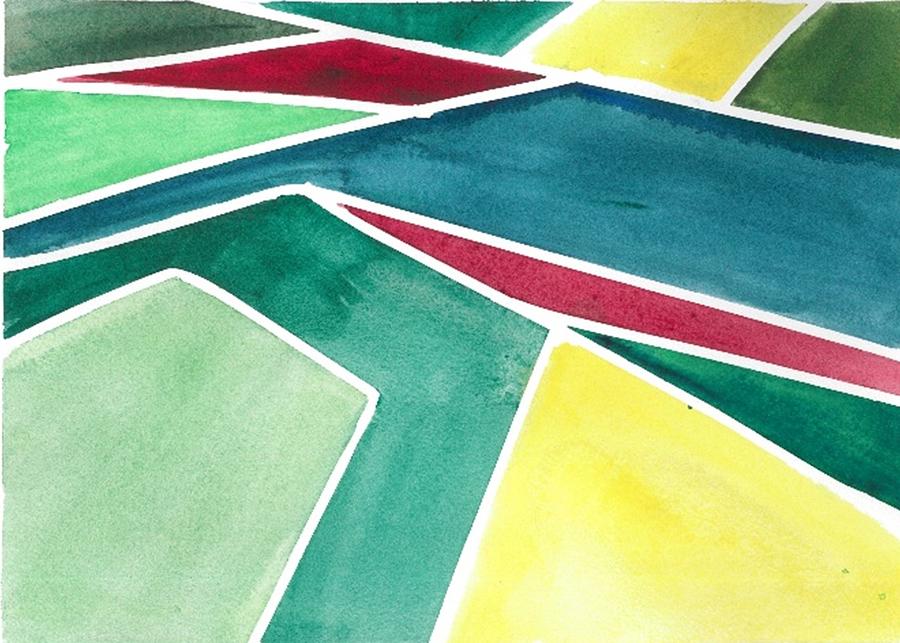The image is a color landscape painting titled "Salt Evaporation Ponds No. 1" by Diane Chen, created in a 1970s retro style. This modern abstract artwork features an array of multi-faceted geometric shapes that are irregular and adjacent to one another, each separated by white borders. The shapes, including diamonds, quadrangles, rectangles, and triangles, are rendered in watercolor-like textures, giving them a fabric or suede appearance. The vibrant palette consists of light greens, aqua, blue, yellow, and deep red hues. These interlocking shapes form a rhythmic pattern, moving diagonally from the top left to the center right of the painting, echoing a distinctive retro aesthetic.